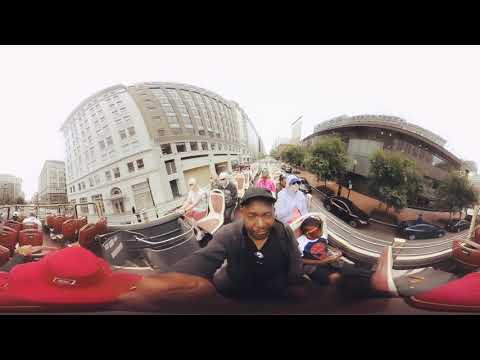This panoramic, 360-degree image captures a bustling urban scene from the top of a double-decker tour bus, where a black man wearing a black hat and black clothes is taking a selfie. The sky appears almost pure white, adding contrast to the cityscape. In the foreground, the seats of the bus are visible, filled with around ten people seated high up. The left side of the image shows a row of empty seats on the bus, with multi-story white and beige buildings in the distance. On the right side, a brown building with a beige wall and some trees stands adjacent to a line of parked cars before the street. The perspective offers a slightly downward view onto the street and cars below. The urban setting hints at a possible location like London, supported by the distinctive double-decker bus. A black border frames the top and bottom of the image, accentuating its panoramic nature.